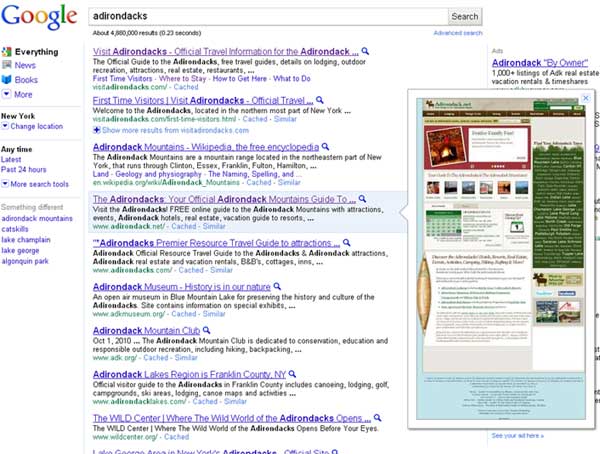This is a detailed screenshot of Google's homepage, captured during a search session. The background is predominantly white, maintaining Google's classic clean aesthetic. 

At the top left corner of the page, the iconic Google logo is displayed in its classic blue, red, yellow, and green colors. Adjacent to the logo on the right is a lengthy search bar, which extends roughly two-thirds of the way across the page. The search bar contains the typed word "ADIRONDACKS" in black font. To the right end of the search bar sits a gray button with the word "Search" in black font.

Immediately below the search bar, there's a link labeled "Advanced options" in blue text. Directly under this, another section appears with the term "ADIRONDACKBYOWNR" in purple text.

A notable feature is a partially obstructed, blurry pop-up tab with a white border overlaying part of the screen, making it difficult to discern its content. 

Below the Google logo, a series of clickable tabs is present. The top tab, marked "Everything" in black, is followed by tabs labeled "News," "Books," and "More," all in blue text. Beneath this set of tabs is a thin horizontal line separating them from the next section.

The next section includes location and time-based search tools. "New York" is displayed in black, accompanied by a "Change location" option in purple. Additionally, there are time filters listed as "Any time" in black, "Latest," "Past 24 hours," and "More search tools" in purple.

Finally, under the main search bar, there are ten clickable links with purple titles; each link has additional information in black lettering underneath. Notably, the fourth link down features a light blue border surrounding it, highlighting it among the other results.

Overall, the screenshot captures a typical Google search page with various search tools, options, and results detailed in color-coded text.